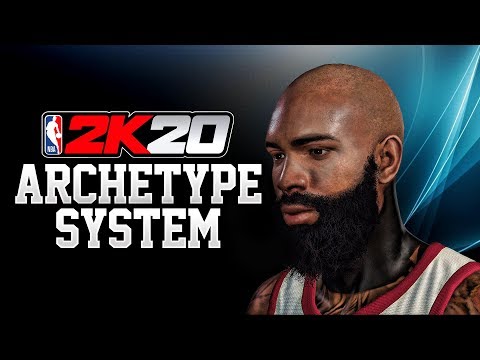This screenshot from the video game NBA 2K20 features a distinctive visual layout, framed by a black border approximately three-quarters of an inch wide at the top and bottom. Prominently positioned in the middle of the left side is the NBA logo, a red, white, and blue silhouette of a basketball player. Below the logo, the game title reads "2K20" in bold red and white text, with "ARCHETYPE SYSTEM" inscribed in large capital white letters underneath.

On the right side of the image, there's a detailed close-up of a virtual basketball player from the shoulders up. The player is dressed in a jersey that can either be red or white, accented by red borders around the sleeves and neck. The avatar features intricate tattoos on the chest and shoulder and is characterized by a long beard, mustache, and a bald head, with the player gazing off to the left towards the lower portion of the image. The background to the right of the player is adorned with light blue lines, evocative of neon lights, adding a futuristic and dynamic aesthetic to the scene.